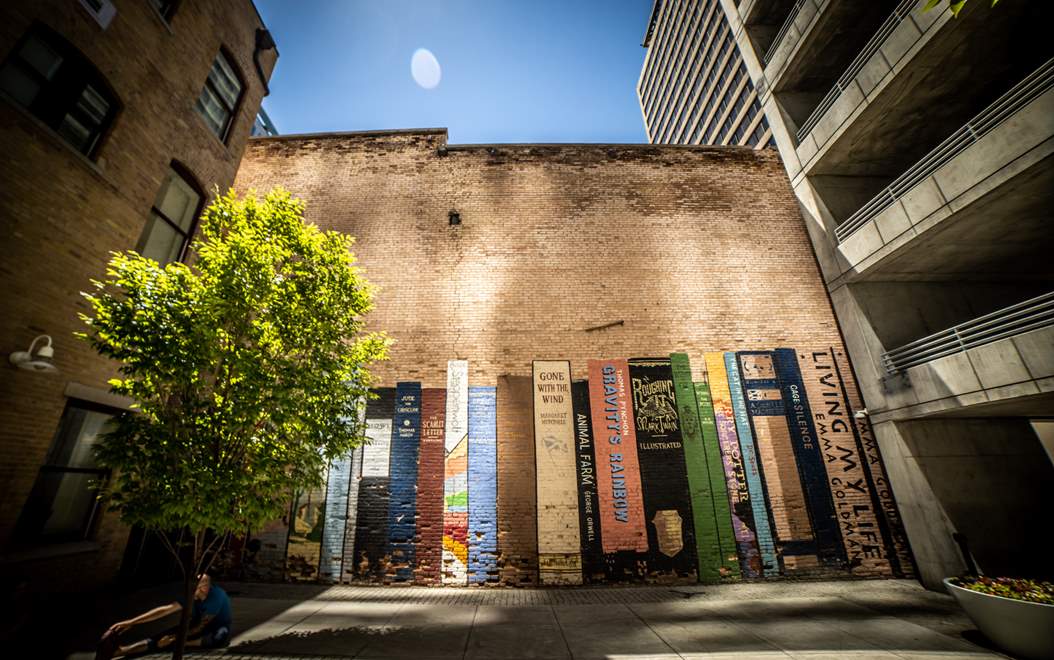The photograph captures a small urban courtyard flanked by towering buildings on either side. To the right stands a tall, white and gray parking garage, while the left features a dark brown brick apartment building. At the center, there's a beige, two-story brick building adorned with a colorful hand-painted mural designed to resemble a bookshelf. The mural consists of numerous books painted spine-out in various colors, including orange, black, green, dark blue, white, and tan, creating the illusion of a densely-packed shelf. Some titles are discernible, such as "Gone with the Wind" and "Living My Life" by Emma Goldman, though many are obscured. A small green tree, approximately 12 feet tall, is stationed to the left of the mural-covered wall. The photo, taken from a paving-stone courtyard, captures a clear, mid-afternoon sky, with a partially visible moon hovering above.